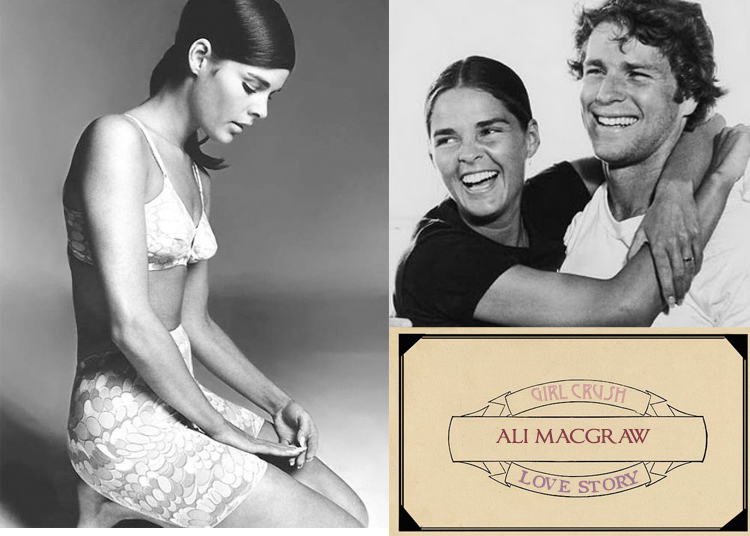This image collage prominently features three distinct photos. On the left, a black-and-white image captures Allie McGraw in a white, scale-patterned bra and skirt or shorts, barefoot and with her hair in a ponytail resting on her left shoulder. She is kneeling and looking down at her hands, which are held just above her legs. The background is neutral and out of focus. The upper right photo shows Allie McGraw again, this time in a black shirt, smiling, and with her arms around actor Ryan O’Neal, who is wearing a white shirt. Both are looking off into the distance with smiles on their faces. The lower right section contains a beige box with a hand-drawn ribbon design and text that reads, "Girl Crush Allie McGraw Love Story" in various colors: "Girl Crush" in pink, "Allie McGraw" in red, and "Love Story" in purple or blue. This combined layout creates a nostalgic, romantic-themed collage centered around Allie McGraw.